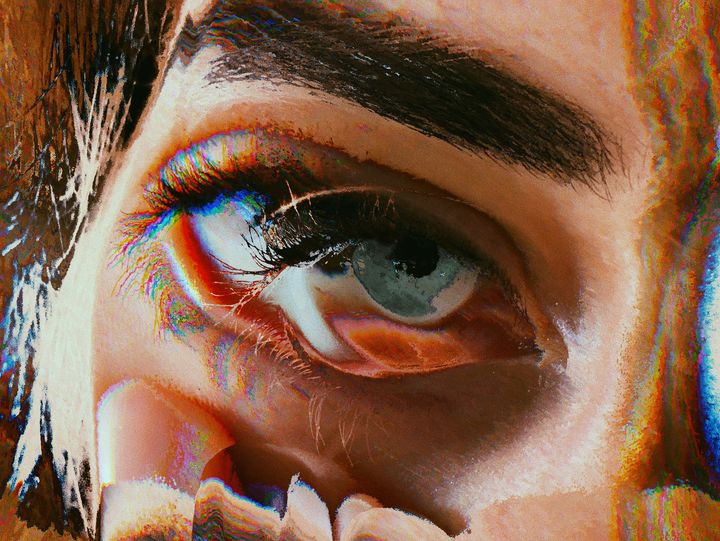The image is an abstract art piece focusing on a close-up of a distorted eye and surrounding facial features. The primary eye, with its sea blue color and long lashes, is strikingly detailed, and behind it, a second eye seems to fade into view, creating an illusion of two eyes merging into one. The prominent, dark brownish-black eyebrow arches dramatically above the eyes, contributing to the surreal effect. The surrounding hair, dark brown with streaks of blue, cascades down the left side of the image, interspersed with hints of fingers possibly pulling at the eye, adding to the bizarre and unsettling nature of the piece. Red tones around the eye area and the partial view of the nose and nose bridge on the right further accentuate the distortions, emphasizing the eye as the focal point in this modern, possibly AI-generated or digitally altered, artistic installation.